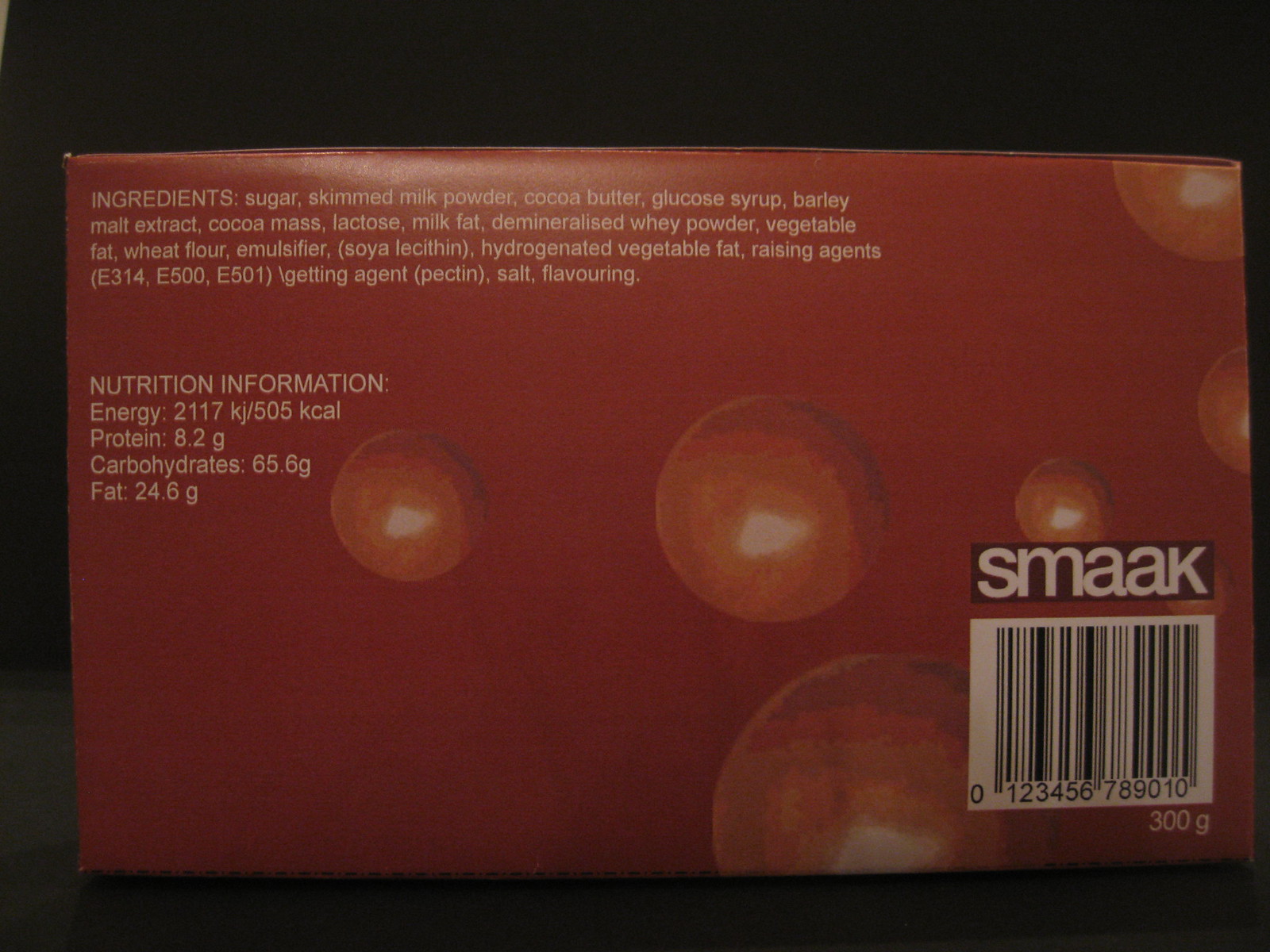This photograph captures a close-up view of a red cardboard box in a dark room, where the background fades into an impenetrable black void. At the bottom edge of the image, a dark-colored table surface is barely visible. The red box occupies most of the frame and prominently displays the logo "SMAAK" in white letters. A white barcode stripe with black lines and "300 grams" noted below it is also visible. The box is adorned with several round orange balls, some with a yellow blotch in the center. These balls vary in size and are distributed across the box's surface, with the largest one partially cut off at the bottom edge of the image. An ingredients list, printed in white, lists various components like sugar, skim milk powder, and cocoa butter, among others, followed by detailed nutritional information including energy, protein, carbohydrates, and fat contents. This text is centrally placed on the box’s surface. The entire box is framed by a stark black background, accentuating the rich maroon shade of the packaging.